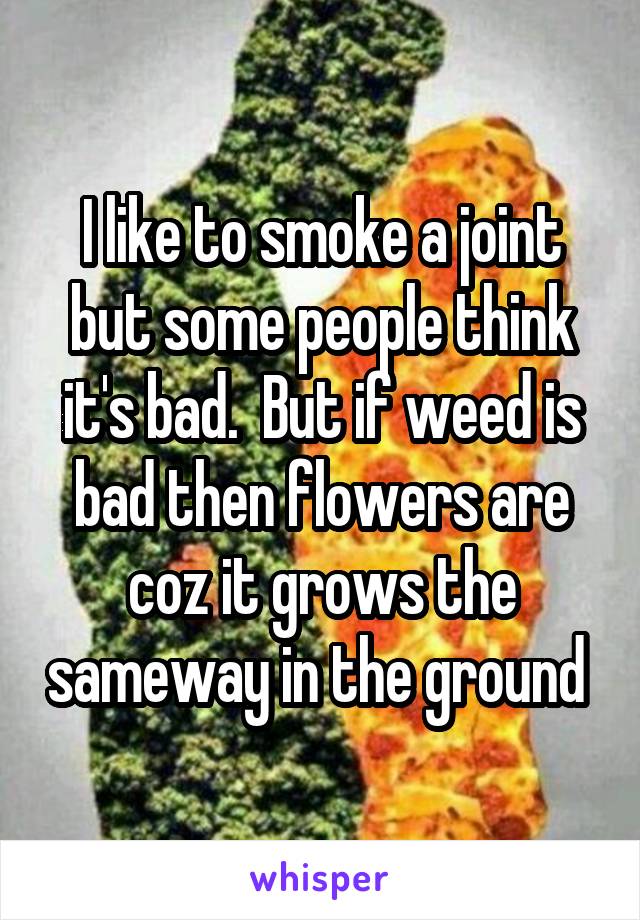The poster features a gradient gray background transitioning from darker gray at the edges to almost white towards the center. At the center of the image, two silhouetted figures are depicted - a man on the left formed out of marijuana leaves and a woman on the right, with an ambiguous texture that some suggest resembles pizza or fire. Both figures are positioned facing each other and are centered both vertically and horizontally within the poster. Above the figures, white bold lettering with a black outline reads: "I like to smoke a joint, but some people think it's bad. But if weed is bad, then flowers are because it grows the same way in the ground." At the bottom of the poster, the word "Whisper" is written in purple, possibly indicating a brand or social media platform associated with the message.